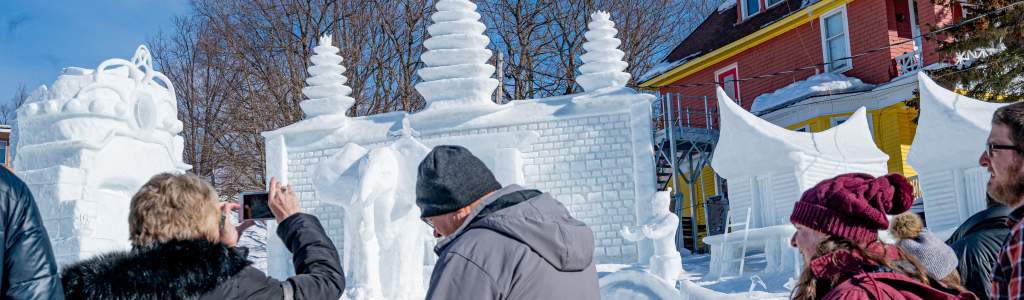This is a detailed photograph featuring a group of four individuals dressed in winter attire, viewing elaborate sculptures crafted from ice and snow. The scene highlights several tall and intricate ice sculptures that resemble buildings, including a house with a ladder, a fanciful hut, and what appears to be a section of the Great Wall of China. One sculpture is topped with elements that resemble trees or fountains. The backdrop includes a red house with yellow and a bit of red trimming, along with bare tree branches under a clear, blue sky. From left to right, the people in the photograph are: an individual whose arm is partially visible, a blonde woman in a gray coat with black fur around the neck holding up a camera, a man in a gray jacket with a gray knit hood, a girl in a red wool hat and red jacket, and someone with glasses and a beard on the far right. The image captures the vibrant and festive spirit of an ice sculpture competition, common in many Midwestern towns.